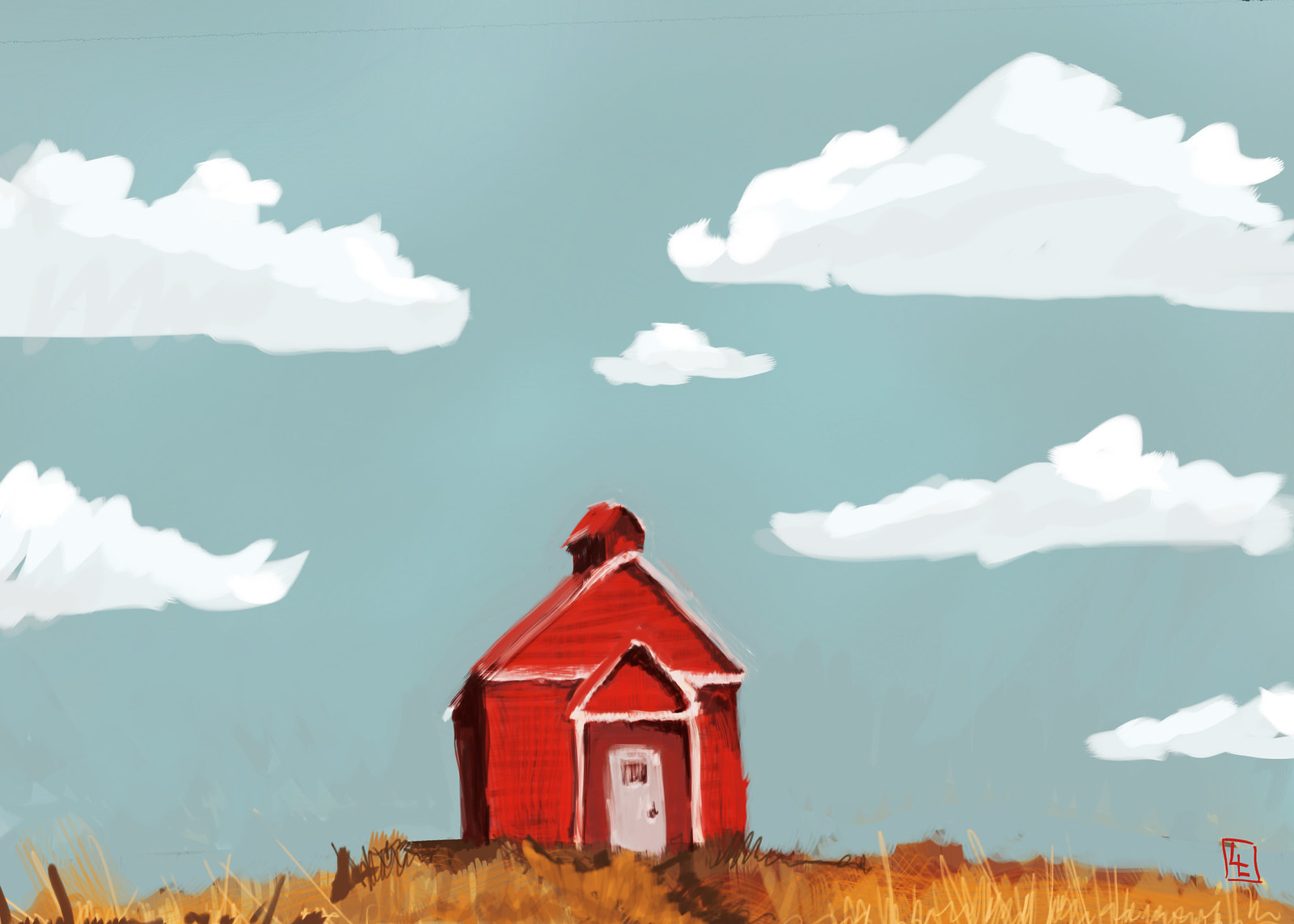This image features a rudimentary landscape painting, characterized by an array of loosely formed, fluffy clouds set against a moderately deep blue sky. The centerpiece of the artwork is a red structure with a white door and a steeple, reminiscent of a church but decorated in the traditional red and white colors typically associated with barns. This building stands in the middle of what appears to be a field composed of hay or dead grass. The painting is signed, though the signature, possibly "ZL," is somewhat unclear.